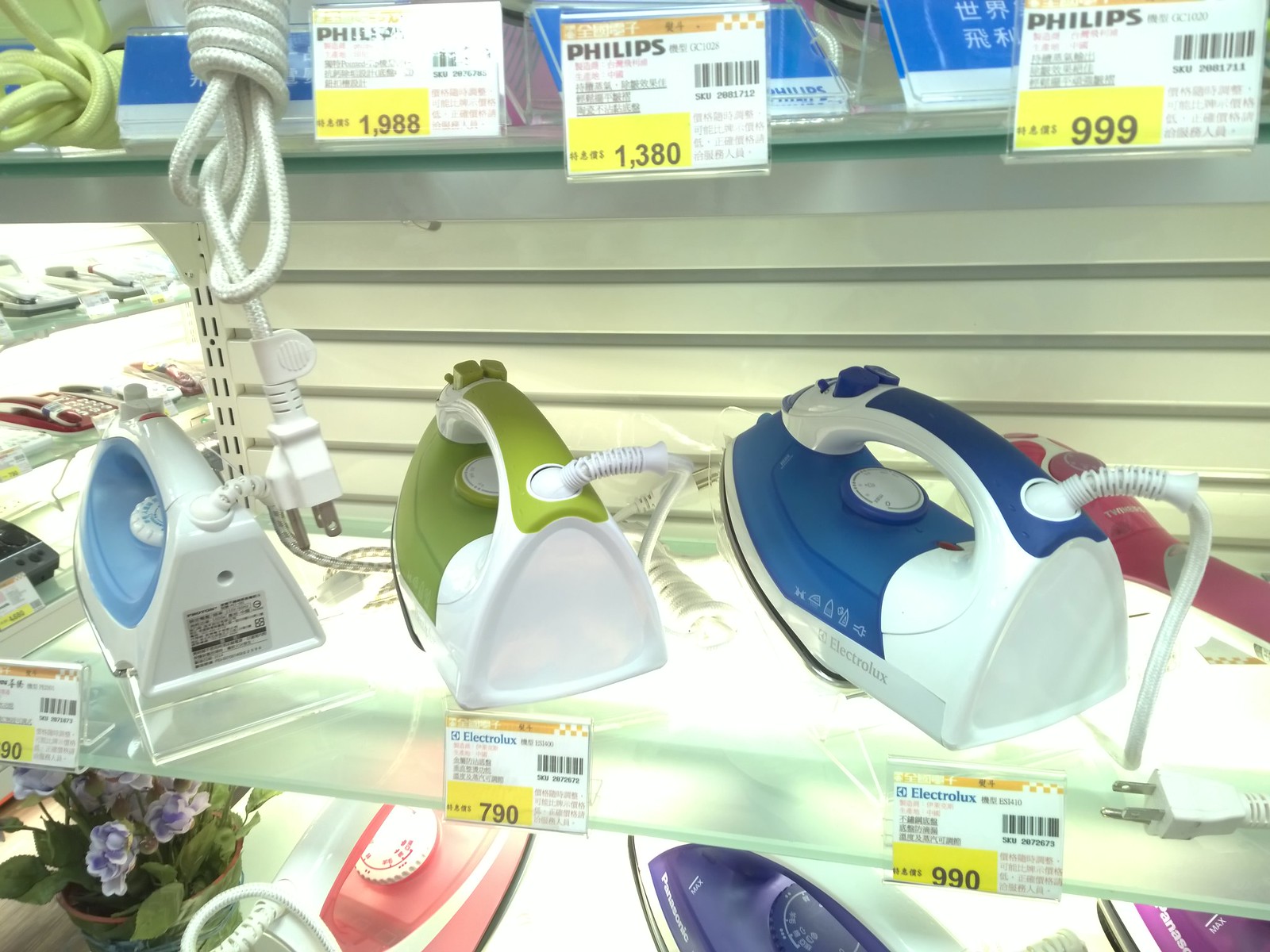This detailed photograph, likely taken inside a department store or supermarket, showcases a display of various Electrolux and Philips clothing irons neatly arranged on two shelves. The middle and bottom racks each hold three irons, featuring an array of colors including light blue and white, dark blue and white, green and white, purple and white, and pink and white. Each iron is marked with a yellow price tag displaying the prices in black text, though only the green and white iron ($7.90) and the dark blue and white iron ($9.90) prices are fully visible. Additionally, there is a noticeable flower vase with purple flowers placed at the bottom left of the bottom shelf, enhancing the display's aesthetic appeal. A Philips logo is prominently visible on the description tags affixed to the middle rack, suggesting a mix of brands within the display.